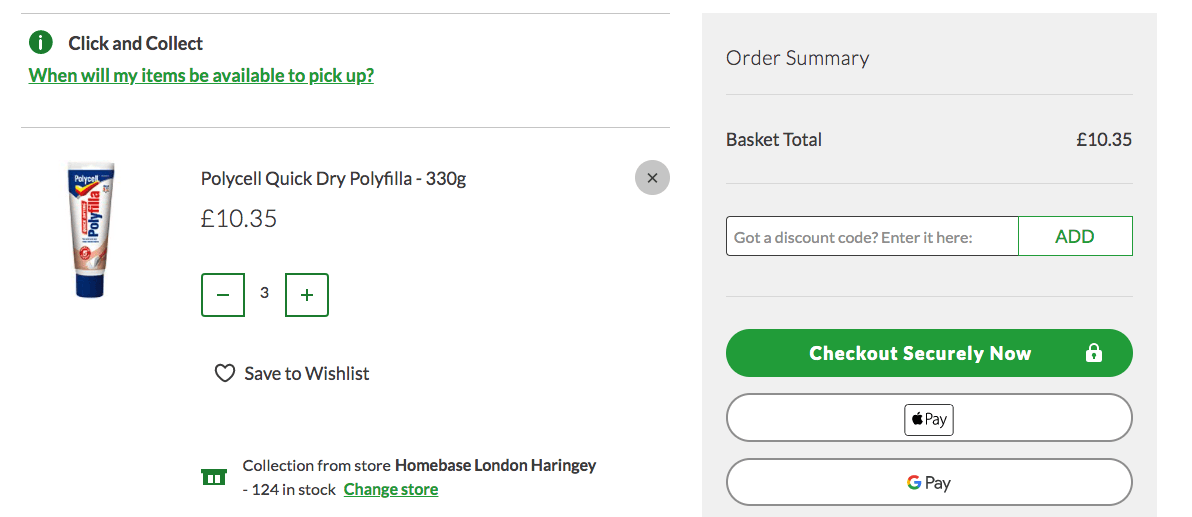This image showcases a detailed order form from an online shopping platform. The form is divided into two main sections:

**Left Section (occupying about 60% of the width):**
- **Click and Collect Information:**
  - A header titled "When will my items be available to pick up?"
- **Product Details:**
  - An image of a Polysil Quick-Dry Polyphia, weighing 330 grams.
  - Price: £10.35.
  - Quantity Selector: A plus and minus option to adjust the quantity, currently set to 3.
  - Save to Wishlist: An icon of a heart with an option to save the item to a wishlist.
- **Store Information:**
  - Collection Point: Homebase London Haringey.
  - Stock Availability: 124 items in stock.

**Right Section:**
- **Order Summary:**
  - Background: Light gray.
  - Font Color: Black.
  - Basket Total: £10.35.
  - Discount Code: A box to enter a discount code with an adjacent 'Add' button.
  - Checkout Options: Three buttons for checkout:
    - Green button: "Check out securely now"
    - White button: "Google Pay"
    - White button: "Apple Pay"

This comprehensive order form provides clear product details, flexible quantity adjustment, and multiple secure checkout options, making the shopping experience user-friendly and efficient.